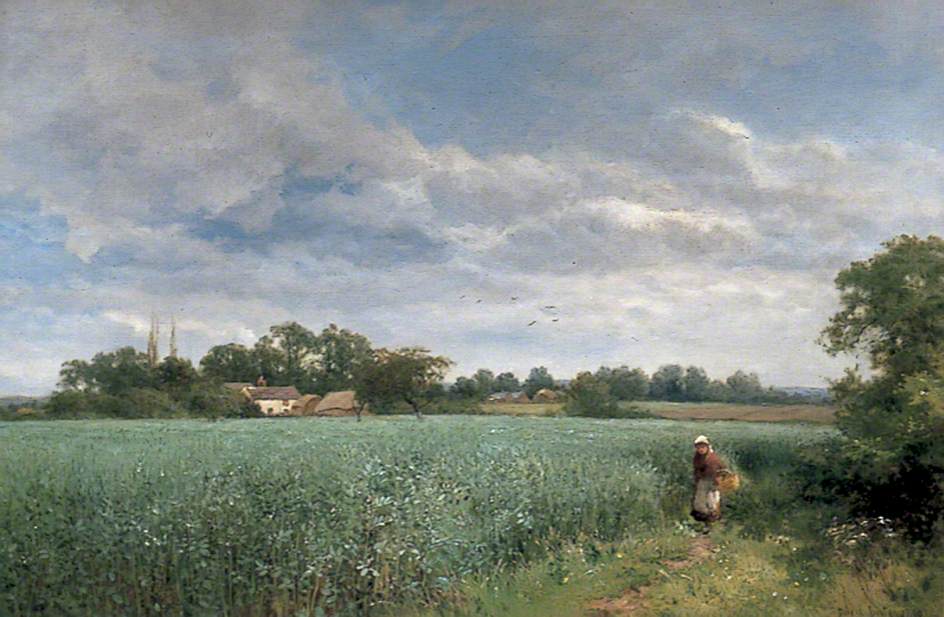This painting is a highly detailed depiction of a sprawling outdoor field, almost lifelike in its intricacy. The foreground is a lush green field dotted with white flowers and sections of shorter grass. Prominently featured in the lower right is a lady in a long, 19th-century-style dress—primarily red with a white headdress and apron—carrying a basket on her left arm. She stands near a large tree filled with green leaves. A dirt path runs alongside the field, leading towards a distant white house with a gray roof, partially obscured by trees. Additional houses can be seen on the horizon, surrounded by more trees. The sky above is a vibrant blue, scattered with white and gray clouds, suggesting daytime. The field stretches on, eventually sloping down and opening up to another expanse, embodying the vast, open landscape of a farm.